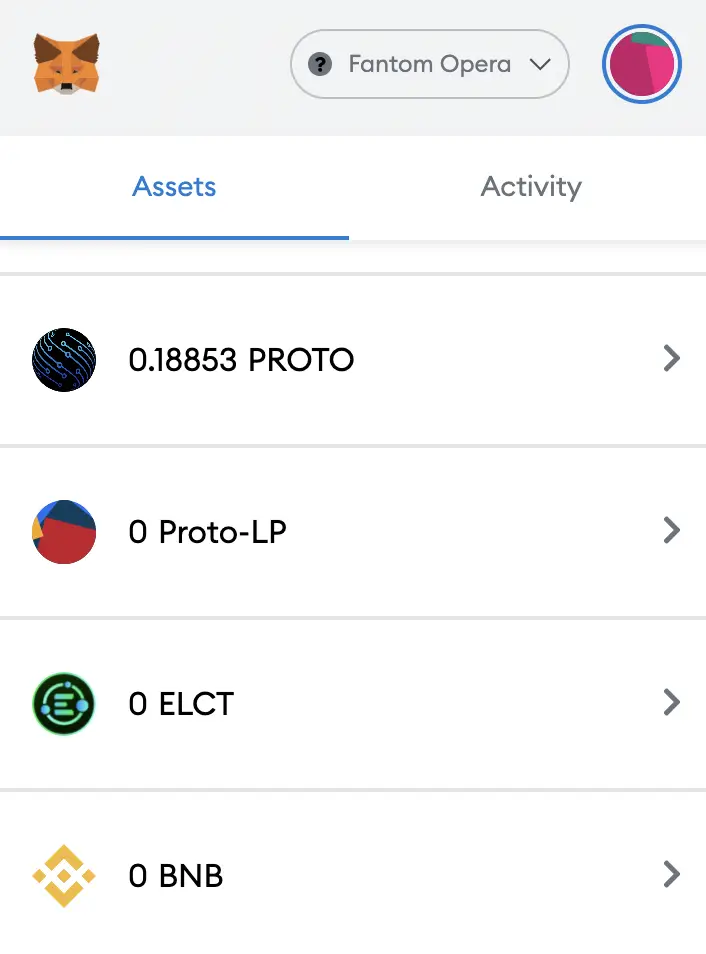Caption: 

The interface displayed is that of a cryptocurrency wallet. The upper 15% of the screen features a light gray background, while the rest of the page is stark white. In the top left corner is a fox icon, symbolizing the commonly recognized crypto wallet. To the right of this icon, "Phantom Opera" is prominently displayed within an oval, accompanied by a small arrow indicating the option to switch accounts or cryptocurrency networks. Further right, a user profile picture is positioned, characterized by a pink hue with a touch of green at the top, enclosed in a blue circle. 

Below this section, the wallet interface is divided into two main tabs. The 'Assets' tab, highlighted in blue and underlined, occupies the left half. The 'Activity' tab, which is gray in color, occupies the right half. 

The main section of the page consists of four individual entries, each representing a different cryptocurrency or token, accompanied by their respective quantities and icons. 

1. The first entry displays "0.18853 PROTO" with an associated icon, and to its right, a gray arrow button.
2. The second entry shows "0 PROTO-LP" alongside its icon and gray arrow.
3. The third entry lists "0 ELCT" with its icon and arrow.
4. The fourth and final entry presents "0 BNB" with an icon and arrow.

Each icon is visually appealing and adds to the overall clean and professional look of the wallet interface.